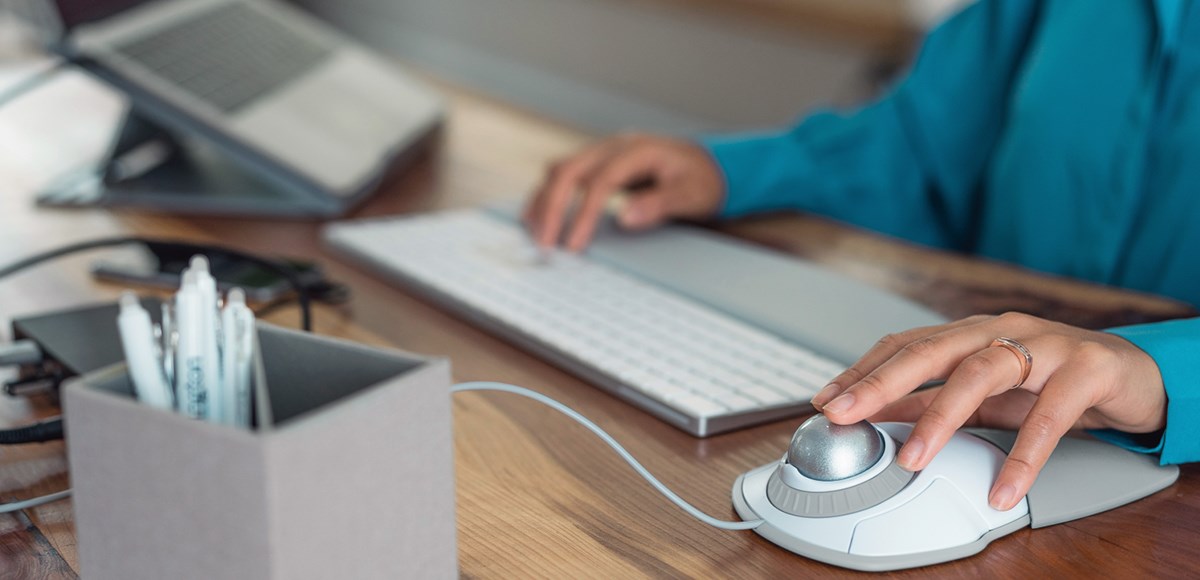This color photograph captures a detailed scene of a woman working at a desk. The focal point of the image is her left hand, adorned with a ring, resting on a large ergonomic mouse featuring a silver trackball. Her right hand is poised over a sleek, low-profile keyboard with white keys and a light gray wrist rest. She wears a turquoise long-sleeve, button-down blouse. The desk itself is light brown wood and holds several items: a small beige pencil case filled with white click pens, a dark cell phone, and what appears to be a laptop propped up in the background. Also visible are a black router with tangled cords and possibly another electronic device. The background is blurred, emphasizing the woman's hands and the immediate workspace while obscuring the rest of the scene.